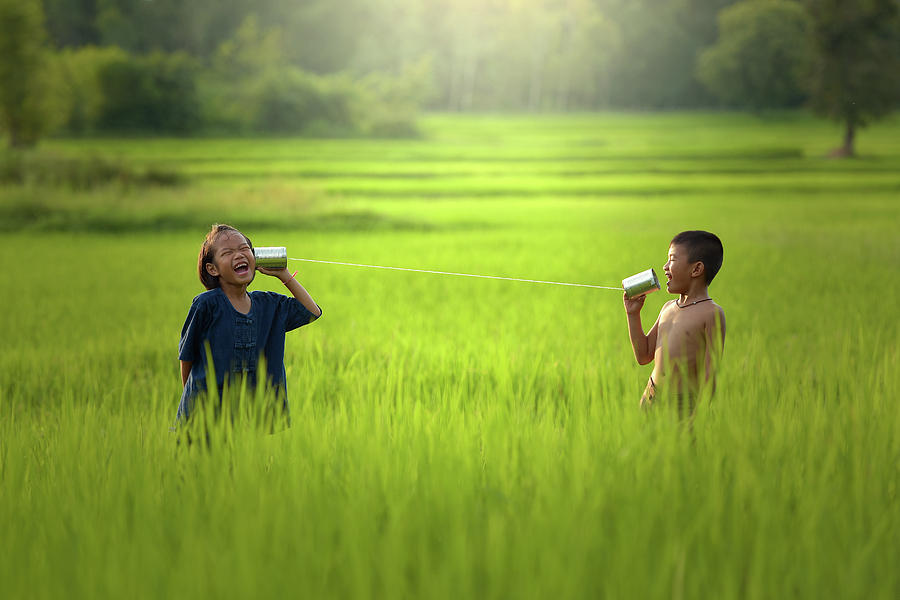In this adorable photograph taken in a sunlit field, two children—likely around seven or eight years old—stand waist-deep in tall, light green grass, creating a scene filled with joy and innocence. The central focus is on a shirtless boy with brown hair on the right, wearing a black necklace, who is speaking into a tin can telephone. This makeshift device is connected by a string to another tin can held by a girl on the left. She has short brown hair, a South Asian racial background, and wears a navy blue top or dress. She holds the can to her ear, laughing at what the boy is saying. The children are captivated by their playful conversation, their smiles radiating happiness. The background is a blur of lush green trees with sunlight peeking through the foliage, casting a natural glow over the scene and emphasizing the carefree atmosphere of their youthful adventure.